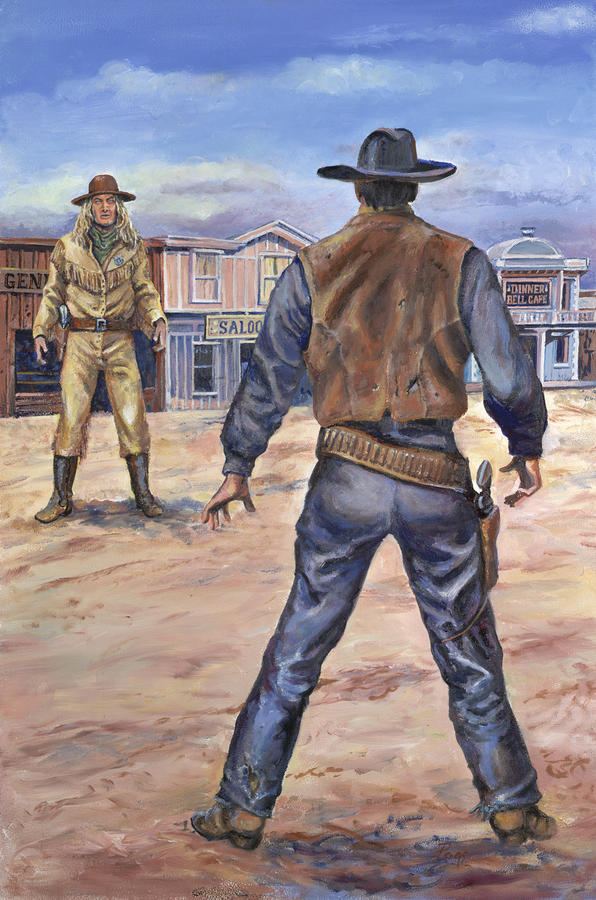This is a detailed colored illustration of a gunfight set in the Wild West. The scene features two cowboys facing off against each other on a gravel or dirt street outside a saloon. The sky is blue with scattered clouds. 

The cowboy positioned at the upper left corner of the image, facing the observer, has long blonde hair and is dressed in a beige outfit over a green shirt or neckerchief, with dark boots and a brown hat. He's poised, with his right hand hovering close to his gun, ready to draw.

The larger cowboy occupies the lower right to upper right portion of the composition, turned away from the observer. He wears a blue long-sleeved shirt under a dark brown leather vest, blue jeans, brown boots, and a black-blue bowler hat. His right hand is also poised near his holster, ready to draw his pistol, while his other hand is splayed out downward.

The backdrop includes classic Wild West elements, with an identifiable "SALOO-" sign suggesting a saloon, a general store behind the smaller cowboy, and a building labeled "Dinner Bell Cafe" visible over the shoulder of the larger figure. The setting captures the tension and anticipation typical of a showdown in a Wild West town.